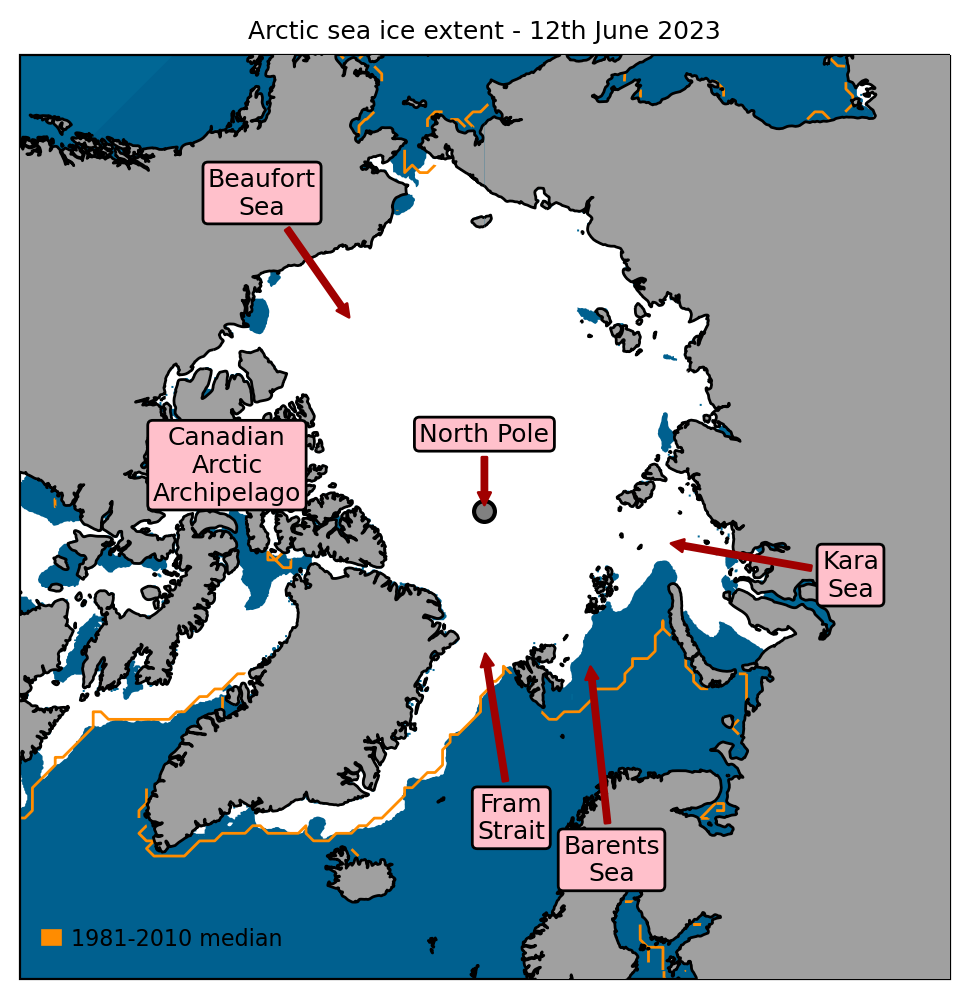The image is a detailed map demonstrating the Arctic Sea Ice Extent as of June 12, 2023, overlaid with a median from the years 1981 to 2010. This drawing distinctly uses gray to color the surrounding sea and landmasses, which notably include parts of North America, Alaska, and Greenland. The central focus is a white area symbolizing the North Pole, marked by a gray dot and a label against a pink rectangular background. Various significant geographic regions such as the Beaufort Sea, Canadian Arctic Archipelago, Fram Strait, Kara Sea, and Barents Sea are labeled with red arrowed lines pointing to their respective locations. These labels are placed within red or pink backgrounds for clearer visibility. Orange lines marking the 1981-2010 median arc across both the top and bottom portions of the map, highlighting the extent of historical ice coverage compared to present conditions. The map employs primary colors of gray, white, and blue for landmasses and sea, emphasizing the changes in ice extent without aiming for realistic satellite imagery.